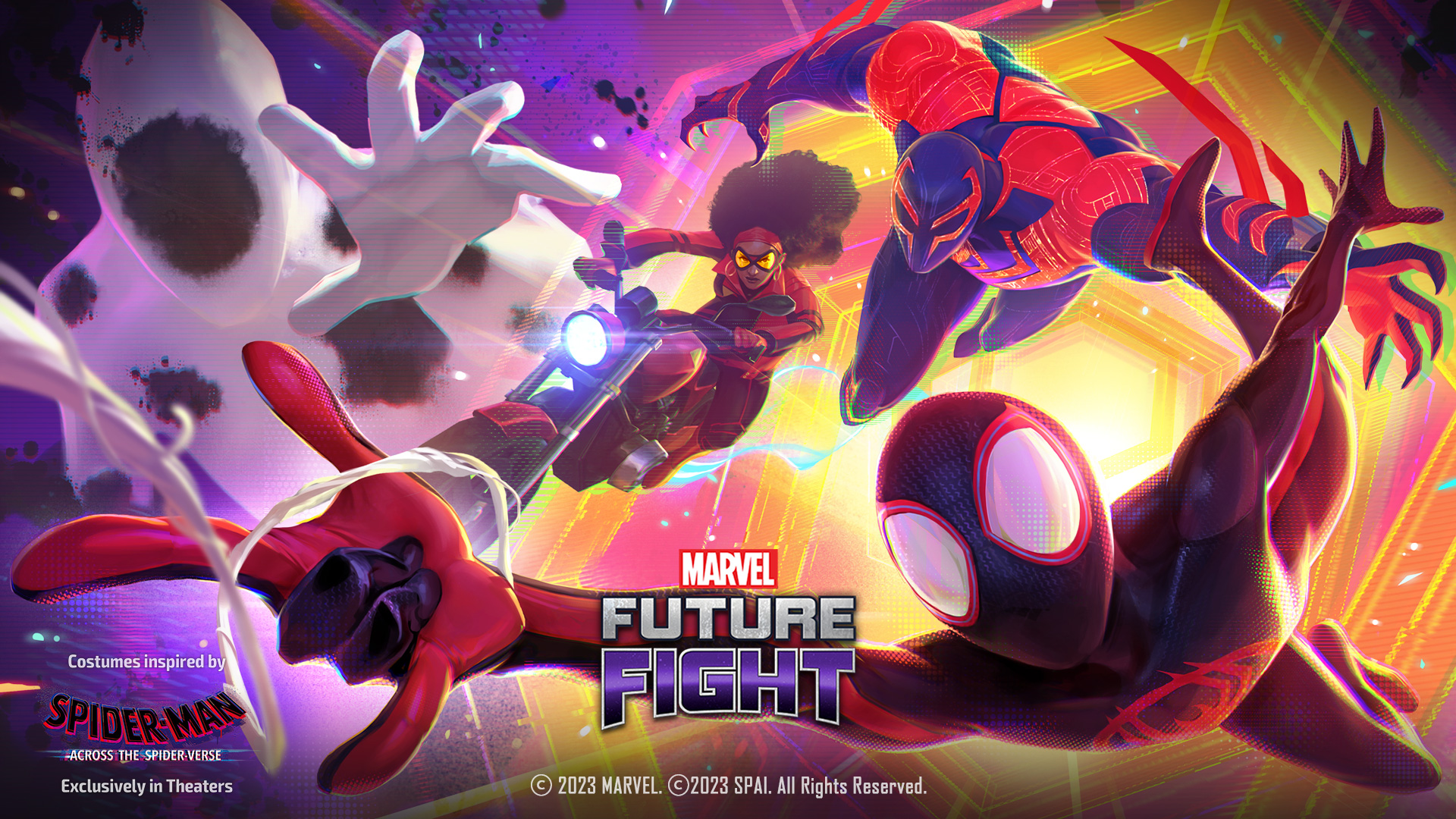This rectangular image, measuring approximately five inches wide by three inches high, serves as an elaborate advertisement for the upcoming Marvel superhero venture, prominently featuring characters inspired by "Spider-Man: Across the Spider-Verse" exclusively in theaters. The backdrop is a vibrant, hexagonal spiral starting small in the center and expanding outward, with yellow at the edges and pink filling the inner sections. 

Dominating the composition are four well-rendered superhero figures. On the lower right, we have Spider-Man, bedecked in his iconic red and black suit, complete with large white eyes and grid-like patterns. His fingers are poised in a classic web-shooting pose, and a stream of web fluid can be seen emerging from his wrist. A few splotches of black are seen around his mask and costume, adding a dynamic flair.

Just above Spider-Man is a second figure in a similar costume, though this one's outfit features claws and blends red and black elements. His pose evokes a sense of combat readiness.

To the left, amidst the hexagonal spiral background, a striking figure in a white suit adorned with black cow-like splotches assumes an aggressive stance. The striking contrast of his costume adds visual interest and breaks up the continuity of warm tones.

In the center, adding movement and energy, is a woman with brown skin and a large, poofy black afro, riding a motorcycle. She dons a fitting costume with sunglasses and commands attention as her red and black vehicle surges through the space.

Text elements anchor the visual narrative: The bottom center reads "Marvel Future Fight" in bold, colorful typography—red and white for "Marvel," transitioning from red to purple for "Fight." Below that, copyright information reads "© 2023 Marvel" and “© 2023 SPAI, all rights reserved." The lower left-hand corner complements this detail, specifying "Costumes inspired by Spider-Man: Across the Spider-Verse exclusively in theaters."

Overall, the image is a vivid and detailed representation blending action, vibrant colors, and promotional text, effectively showcasing the Marvel superheroes and their dynamic realm.